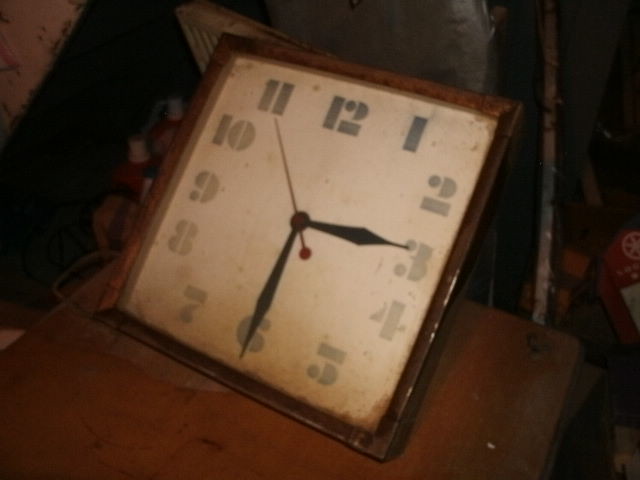The image depicts an old and rusted square-framed clock sitting on a worn wooden tabletop. The clock's frame, once metallic, shows significant tarnish and wear, particularly around the bottom. The clock face, though originally white, has aged and is now dirty. Dark gray, retro-font numbers are arranged in blocks around the face, somewhat faded with time. The bold black hands point to 3:30, while the slender red second hand rests at 11. The setting is dimly lit, casting shadows that further emphasize the clock's age and neglect. In the background, there is a cluttered array of items, suggesting the scene is either an abandoned basement or a dirty garage, contributing to the overall aura of neglect and aging.